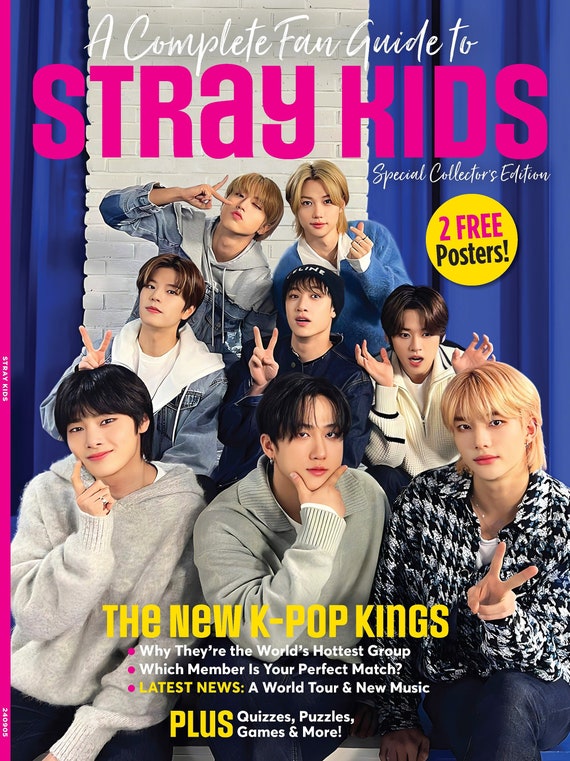The image is a cover of a special collector's edition magazine titled "Complete Fan Guide to Stray Kids." At the top, the headline emphasizes the group's name, "Stray Kids," in bold lettering with the phrase "special collector's edition" beneath it. A prominent yellow circle features the text "Two Free Posters!" Inside the circle, "Two Free Posters!" is written in pink, drawing attention to the added bonus. The cover showcases the eight members of Stray Kids, an Asian K-pop band, all posing and throwing up peace signs in various styles. One member has his fingers positioned around his chin, while another points at his own face. The background includes a white brick wall and blue curtains, adding a cozy, indoor setting to the image. At the bottom of the cover, the phrase "The New K-pop Kings" is highlighted in yellow, along with additional text that reads: "Why They're the World's Hottest Group, Which Member Is Your Perfect Match, Latest News, A World Tour and New Music, Plus Quizzes, Puzzles, Games, and More." The text on the magazine cover appears in vivid colors, predominantly pink and yellow.